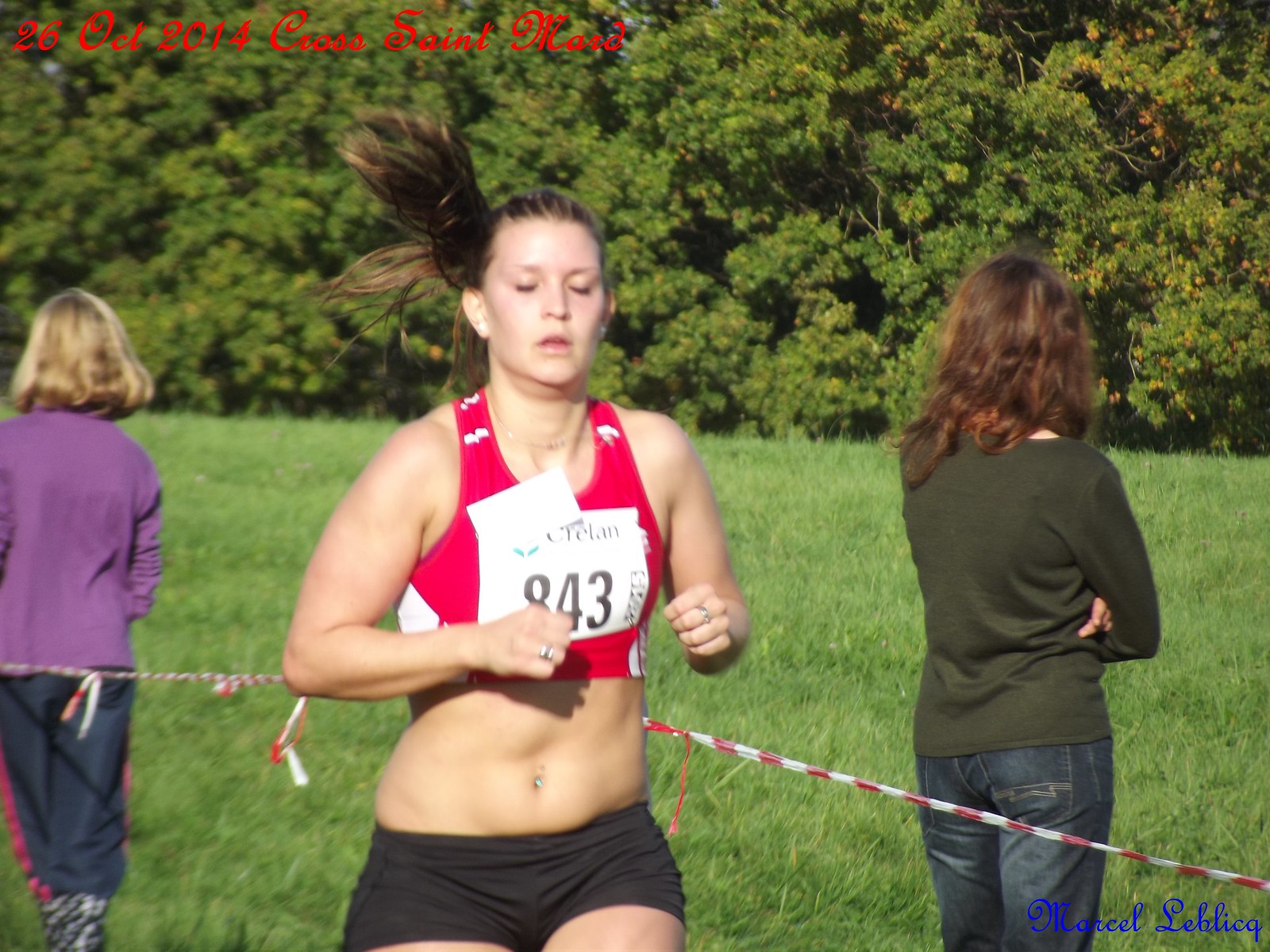In the image, a woman is captured mid-stride as she participates in a race, attired in a black sports bra and black short shorts. Her participant number, 843, is displayed on a small sign pinned to her sports bra. The woman, of white complexion, has her hair tied back in a ponytail that flutters with the motion of her run. Her hands are clenched into fists, and her eyes are closed, suggesting focus and determination. Notable details include a belly button piercing and rings: a wedding ring on one hand and a ring on the middle finger of the other. The background features a field of green grass with two other women, facing away from the camera, standing behind a string fence. One wears a purple long-sleeved top and brown-blue pants, while the other has a dark green top and blue jeans, complemented by long wavy brown hair. Bushy trees with dense green foliage can be seen further back. In the top left corner of the image, the text "26 October 2014, Cross St. Mord" is visible, indicating the event's date and location.